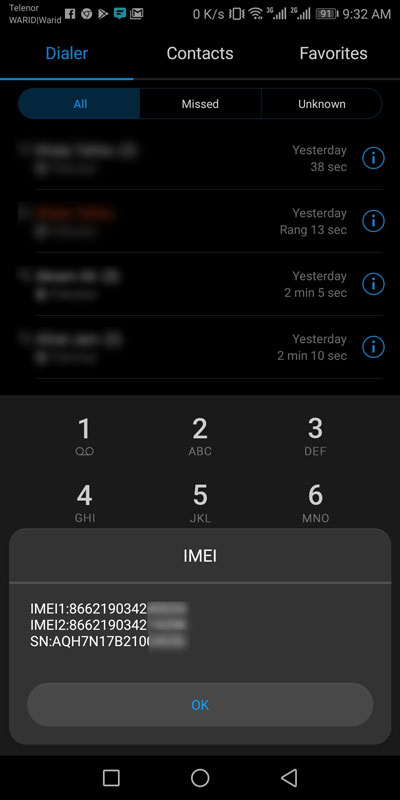The image depicts a smartphone screen showcasing a dialer application interface with a detailed overlay pop-up. At the top of the display, various indicators and icons are visible: 'Telenor', 'Warid', 'Warid' carrier names, a Facebook logo, Chrome, Play Store, chat, and Gmail applications. Network status shows '0k per second' for data, a vibration icon, Wi-Fi signal strength, signal bars for both 3G and 2G, the battery at 93%, and a clock indicating 9:32 a.m.

The main view is a dialer interface where the menu bar includes 'Dialer', 'Contacts', and 'Favorites'. The 'Dialer' tab is highlighted in blue and underlined. The screen is set to display 'All' calls, with categories for missed and unknown at the top. The first four call logs are blurred and illegible. On the right side, timestamps indicate call history: 'Yesterday, 38 seconds ago'; 'Yesterday, 13 seconds'; 'Yesterday, 2 minutes, 5 seconds'; 'Yesterday, 2 minutes, 10 seconds'. Each log entry features a blue information icon ('i' inside a circle).

Beneath the call logs, a numeric keypad for dialing phone numbers is partially obscured by an overlay pop-up. Visible keys include numbers 1 through 6. The overlay displays three lines of alphanumeric text labeled 'IMEI', although the last 20% of this text is grayed out. An 'OK' button is situated below the alphanumeric strings. At the bottom of the screen, a navigation menu bar is partially visible.